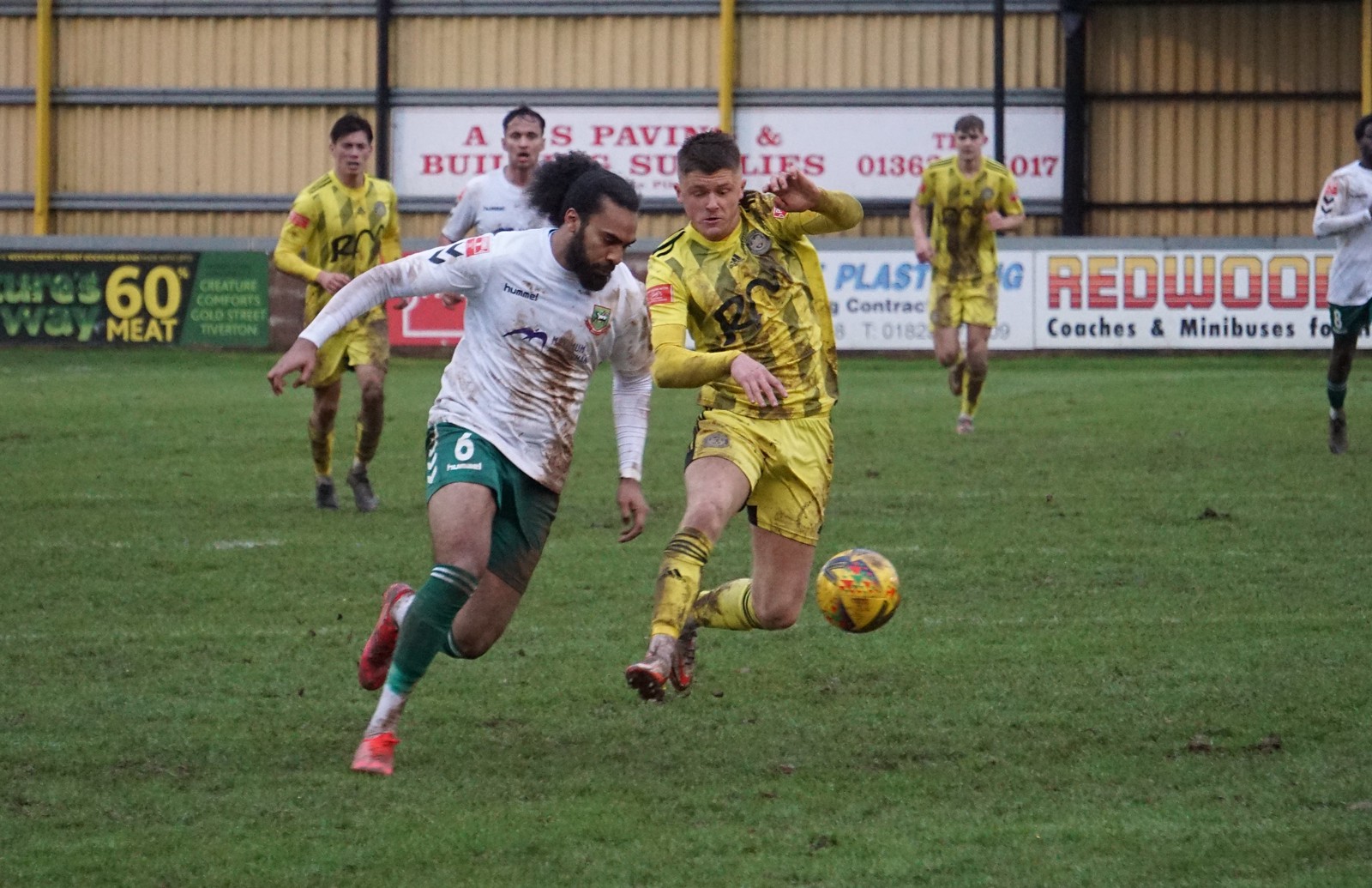In the foreground of a vivid green field with faint white lines, two men are intensely chasing a yellow soccer ball marked with black stains, which is positioned just bottom right of the center. The man on the right is dressed in a yellow soccer outfit with black stripes and stains, complemented by vibrant red shoes. He has short black hair and is gesturing with one hand up and the other down. Beside him, on the left, is a bearded man in a dirt-stained white long-sleeved shirt, green shorts featuring the number six, green socks, and red shoes. His black hair is tied back in a ponytail. In the background, four additional players can be seen: one in a yellow jersey on the far left, another near him in a white jersey, and two more to the right—one in a yellow jersey and the other, an African American man in a white jersey—against a backdrop of banners advertising "Redwood Coaches and Minibuses" on a corrugated steel wall upheld by black and yellow poles. The field, though well-maintained, shows signs of active play with a few divots scattered across its surface.